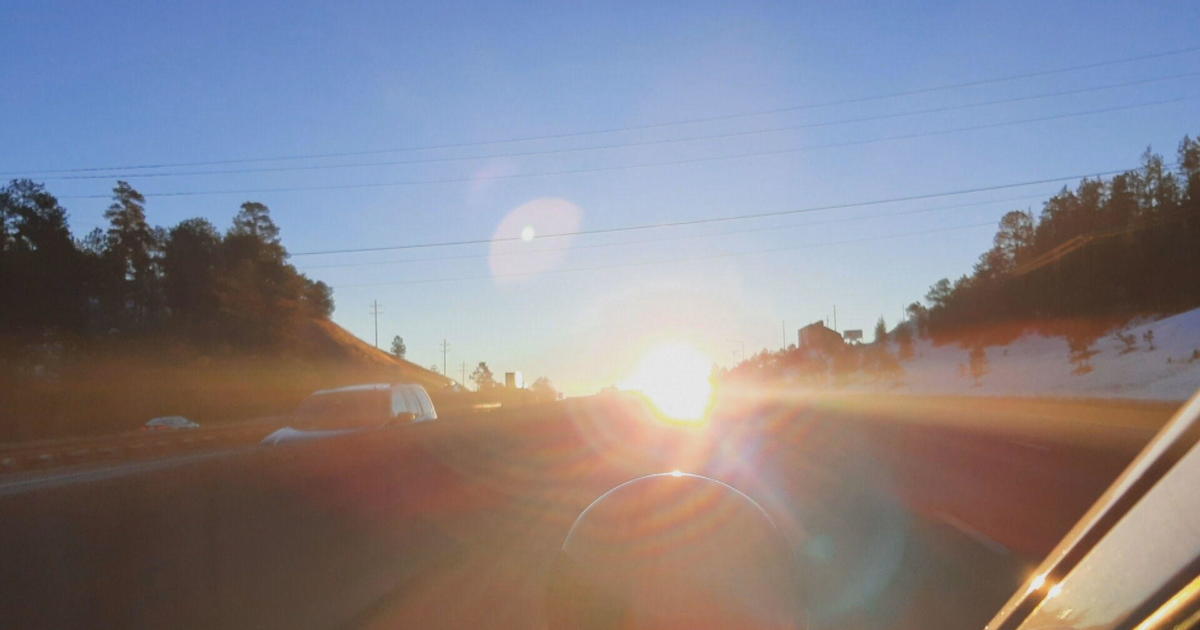This color photograph, likely taken from a vehicle's dashboard camera, captures an outdoor scene along a two-lane highway, potentially during sunrise or sunset. The blinding sun in the center of the image, casting a bright yellow glare, makes it almost impossible to discern the road clearly. The highway is bordered by a snowy landscape and tall trees on either side, suggesting a forested area. On the right side of the road, there is a building in the distance, while a hillside adorned with trees and a line of power poles rises in the background to the left. A barrier separates the lanes of traffic, and another car, possibly an SUV, is visible on the opposite side, moving in the opposite direction. The blue sky tops the scene, adding a contrasting hue to the photograph. Additionally, the interior details of the vehicle from which the image is taken, including a part of the dashboard and the driver's side mirror, are visible in the foreground.